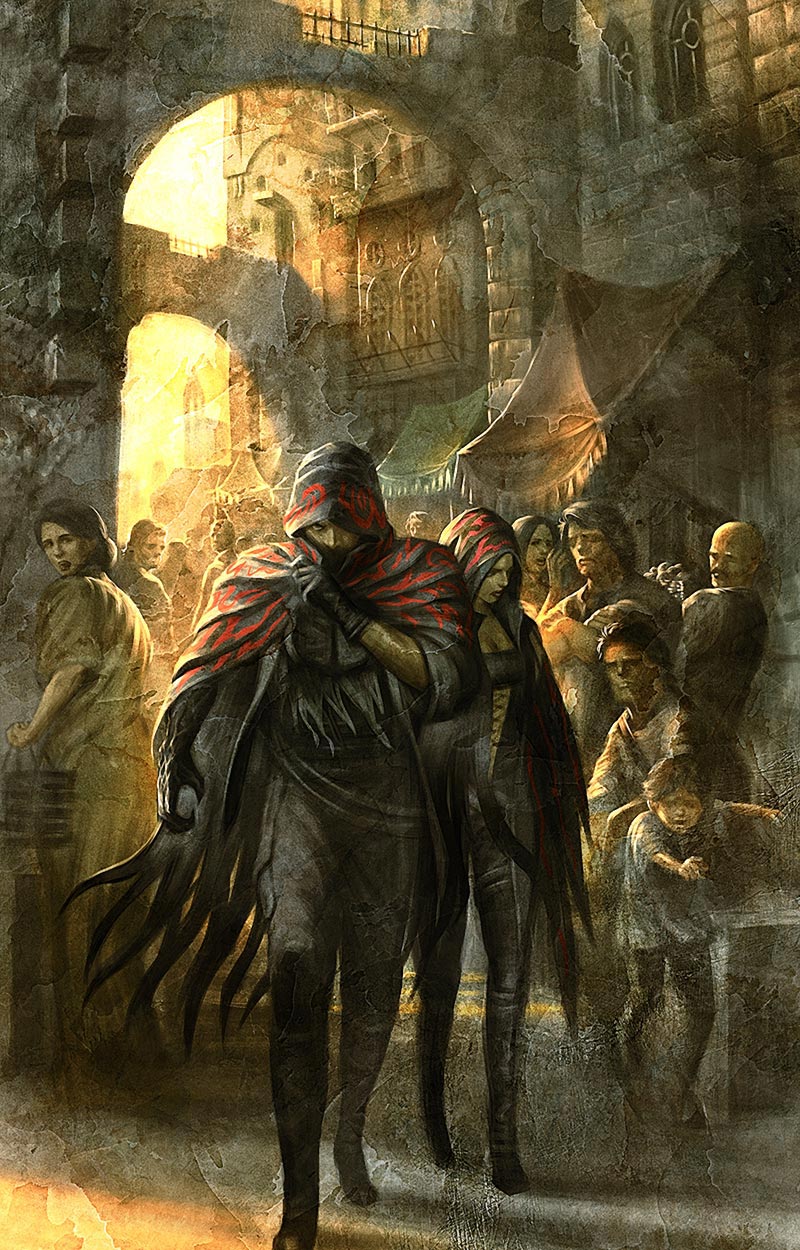In the center of this richly detailed, medieval scene, two imposing figures clad in nearly all-black clothing, accented with red markings around their hoods, stride purposefully through the heart of a bustling, terrified crowd. To the left is a man, his cowl raised to obscure his mouth, giving him an air of mystery and menace. To the right, his female companion mirrors his dark attire and determined expression. Both wear tight leather outfits that exude a dangerous, stylish aura, contrasting sharply with the simpler, dirt-streaked garb of the onlookers around them. The man's claw-like right hand hints at a possibly supernatural nature, further separating them from the ordinary populace. Although the background, with its muted browns, golds, and shafts of sunlight, suggests a medieval castle setting, the sharp focus and distinct style of these central characters make them appear almost out of place, as if from another, more modern era. The scene is reminiscent of a game design or a vivid book illustration, capturing a moment fraught with tension and fear.